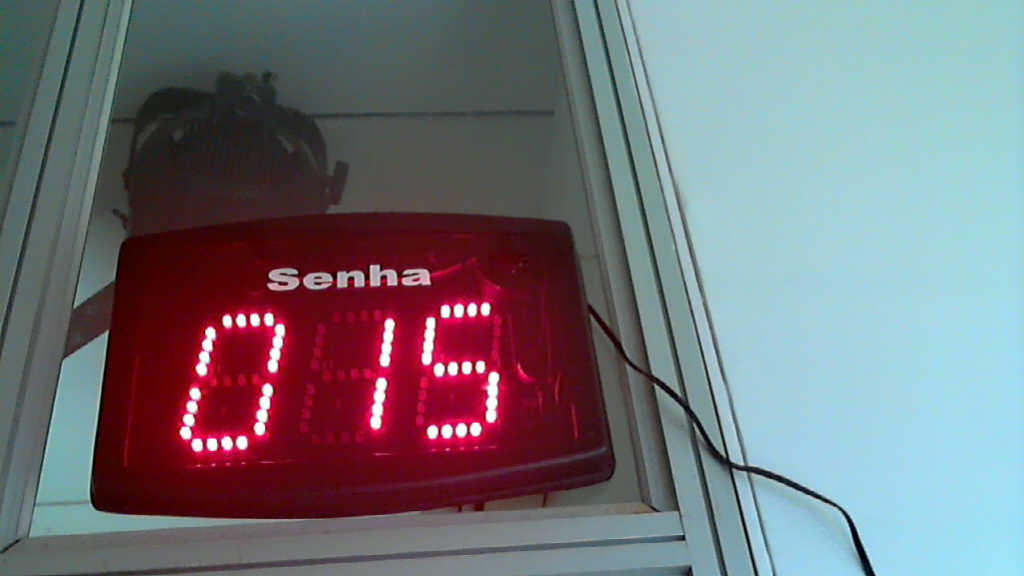A digital display device is prominently featured in this rectangular image. The device itself is square-shaped and predominantly black, with a clear, clean design. Centrally positioned on the display is the word "Senha" in uppercase white letters, which is a Portuguese term for "password" or "number." Directly beneath this word, the number "015" is displayed in a vibrant red digital font, signaling it as the current serving number. The right side of the device includes a connected black cord trailing down to the bottom right corner of the image. The backdrop of the image consists of a plain white wall, providing a stark contrast to the black device. Additionally, a subtle gray frame encompasses the entirety of the device, adding a touch of definition to the overall presentation.